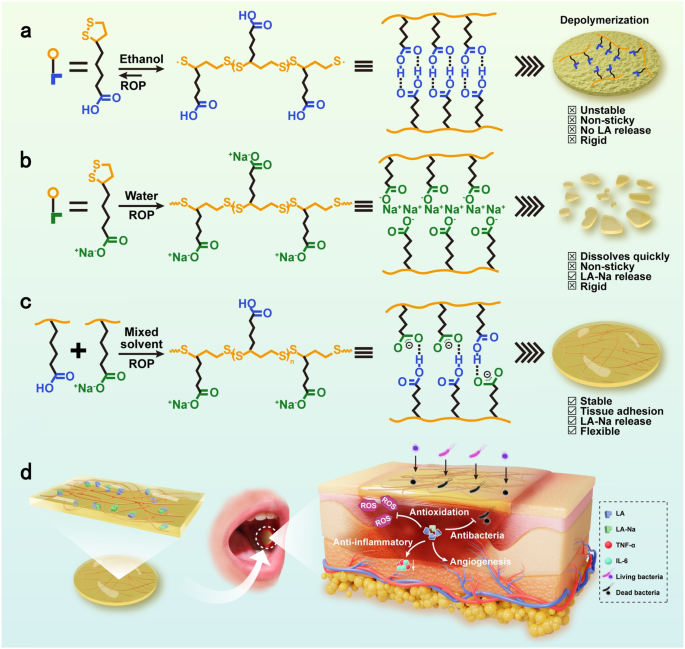This is a detailed, colored diagram, resembling a textbook illustration, featuring a series of chemical reactions and biological processes. The diagram is organized with letters A to D from top to bottom on the left side. Each letter corresponds to a horizontal set of chemical reactions or biological interactions depicted using various chemical formulas and symbols. 

- **Line A**: Features the conversion of ethanol with ROP (ring-opening polymerization) resulting in products with carbon atoms, hydroxyl (HO), and other symbols. The end products are described as depolymerized, unstable, non-sticky, with no LA (likely lactide) release, and rigid.
  
- **Line B**: Illustrates a reaction involving water and ROP, leading to a breakdown that dissolves quickly. The outputs are non-sticky, release both LA and NA (possibly sodium acetate), and remain rigid.
  
- **Line C**: Shows a mixed solvent undergoing ROP. This line's products are stable, exhibit tissue adhesion, release LA and NA, and are flexible.
  
- **Line D**: Depicts a more specialized set of biological photographs related to biological processes and reactions such as anti-oxidation, anti-inflammatory, anti-bacterial functions, and melanogenesis. It involves visual elements like makeup and a mouth, emphasizing the practical applications in biological contexts.

A legend or key is provided at the bottom of the image to clarify the symbols and reactions. This diagram collectively illustrates detailed chemical and biological processes, emphasizing the transformations from one state to another and their respective properties and biological implications.